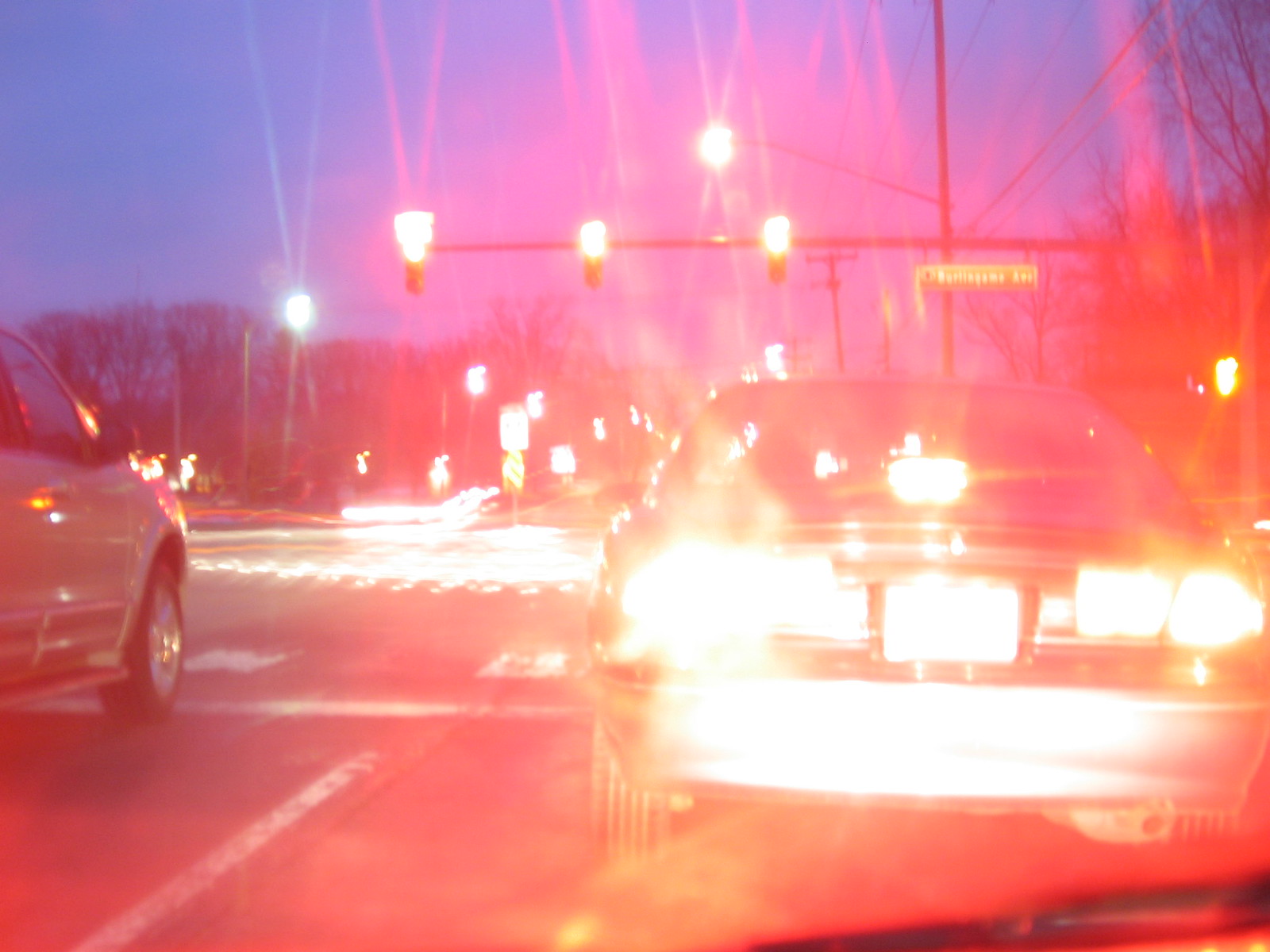The photograph depicts a bustling city street at night, as seen from inside a vehicle. The viewpoint captures the rear end of a light-colored SUV directly ahead and a partial view of a dark-colored sedan to the front-left. Both cars appear to be stopped at a traffic light, possibly red, although the flash from the photo has distorted the color, rendering the lights as bright white with red streaks emanating from them. The street is well-lit by multiple light fixtures and street lamps, which are casting sharp, angular streaks upward into the sky, enhancing the blur effect in the image. A green street sign with white letters, likely indicating the street name and a number, is visible in the distance. The evening sky is tinged with blue, suggesting the photo was taken between late evening and night. Tree outlines can be seen in the background, adding to the urban atmosphere of the image. The intense lighting within the frame affects the visibility of certain details, such as the sedan color and license plates, contributing to the overall blurriness of the image.